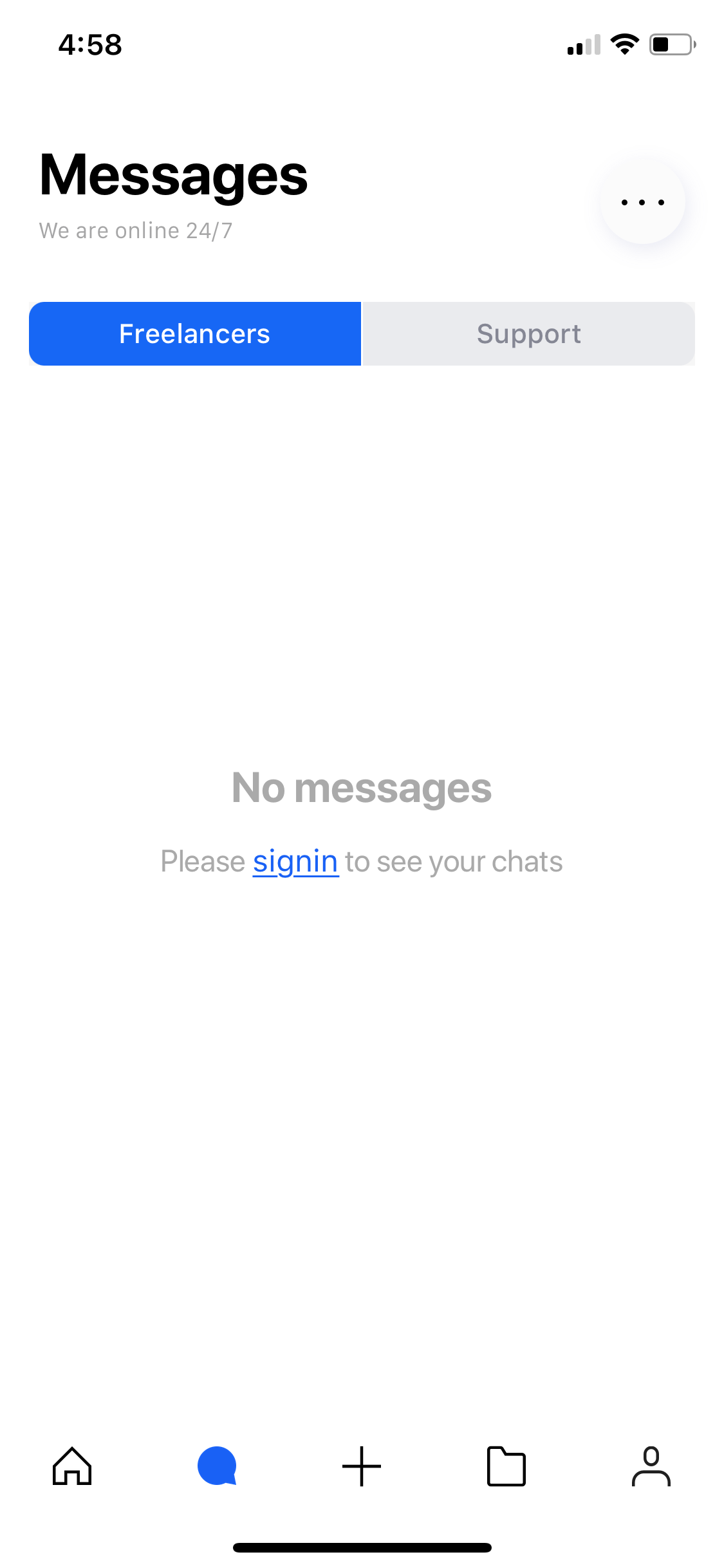This screenshot captures the Messages tab within a mobile app, which is highlighted at the top with the word "Messages" in bold black lettering. Immediately beneath it, in smaller grey text, the phrase "We are online 24/7" is displayed. Two buttons are positioned just below this text: "Freelancers" on the left and "Support" on the right, with "Freelancers" highlighted in blue to indicate it's currently selected. 

Below these buttons, the main portion of the screen is predominantly empty, save for the centered phrase "No messages" in grey print. Further down, in very small grey text, it advises "Please sign in to see your chats," with "Sign in" written in blue and underlined, suggesting it is a clickable hyperlink.

At the bottom of the screenshot, there is a navigation panel consisting of five icons: "Home" on the far left, "Chat" next to it, a centered "Plus" icon, a "File Folder" icon towards the right, and a "User Profile" icon on the far right. 

Other notable elements include the device-specific icons situated at the top of the screen. On the left, the current time is displayed, while the right side shows a series of icons representing phone signal strength, Wi-Fi connectivity, and battery percentage.